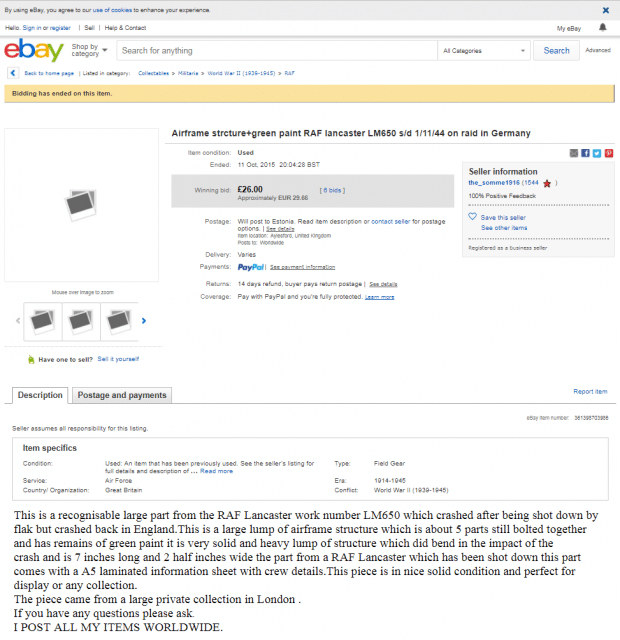The image depicts a screenshot of an eBay webpage with numerous interactive elements and informative text. 

At the very top, a thin gray banner spans the width of the screen with a message stating, "By using eBay you agree to our use of cookies to enhance your experience." The phrase "use of cookies" is highlighted in blue text, contrasting with the black text of the rest of the message. On the far right of this banner, there is a blue 'X' indicating an option to close the notification.

Below the banner, the header includes text that says, "Hello, Sign in or Register." Both "Sign in" and "Register" are in blue print. Following this, there's a vertical line separator, after which the options "Sell," another vertical line, and "Help & Contact" are listed. On the far right side of this section, there's a dropdown menu labeled "My eBay" accompanied by a bell icon.

Further down, the main navigation bar indicates "eBay Shop" and "Shop by Category," the latter having a dropdown arrow for more options. A prominent search bar takes center stage with the placeholder "Search for anything," and a dropdown menu stating "All Categories." To the right side of the search bar, there is a blue "Search" button. Adjacent to this is an "Advanced" search option.

Underneath the search bar, a smaller blue box with a left-pointing arrow includes the text "Back to homepage" in blue print. The next section says "Listed in category" in black text; however, the category text itself is blurred and unreadable but appears in blue.

Proceeding further down, a yellow banner alerts that "Bidding has ended on this item." Below this banner, there is a placeholder image, depicted as a square with Polaroid pictures, indicating the absence of an actual product image. Information regarding the product details and its worth appears beneath this placeholder image.

Overall, the screenshot portrays a detailed view of an eBay product page, complete with navigational elements, notifications, and a partially obscured item listing.